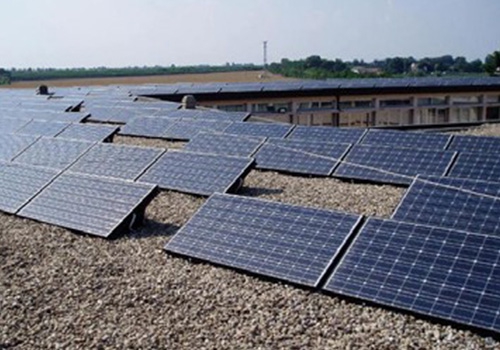The image showcases an array of solar panels positioned diagonally on the gravel-covered roof of a building. The solar panels, square and rectangular with a grid of white lines against dark gray and blue surfaces, are strategically angled to maximize sunlight exposure. They stretch from the bottom right to the center of the image, mounted on stands at a slight tilt. The roof is scattered with loose stones, enhancing the utilitarian aesthetic of the setup. In the background, we see the long, narrow facade of the building extending towards the top right, with additional solar panels visible atop its surface. Beyond the building, a light blue sky, a distant tree line, and open fields come into view. Shadows formed by the panels suggest that the sun is positioned to the left and slightly above the scene. The overall image is devoid of text, allowing the focus to remain on the solar panel installation and its surroundings.